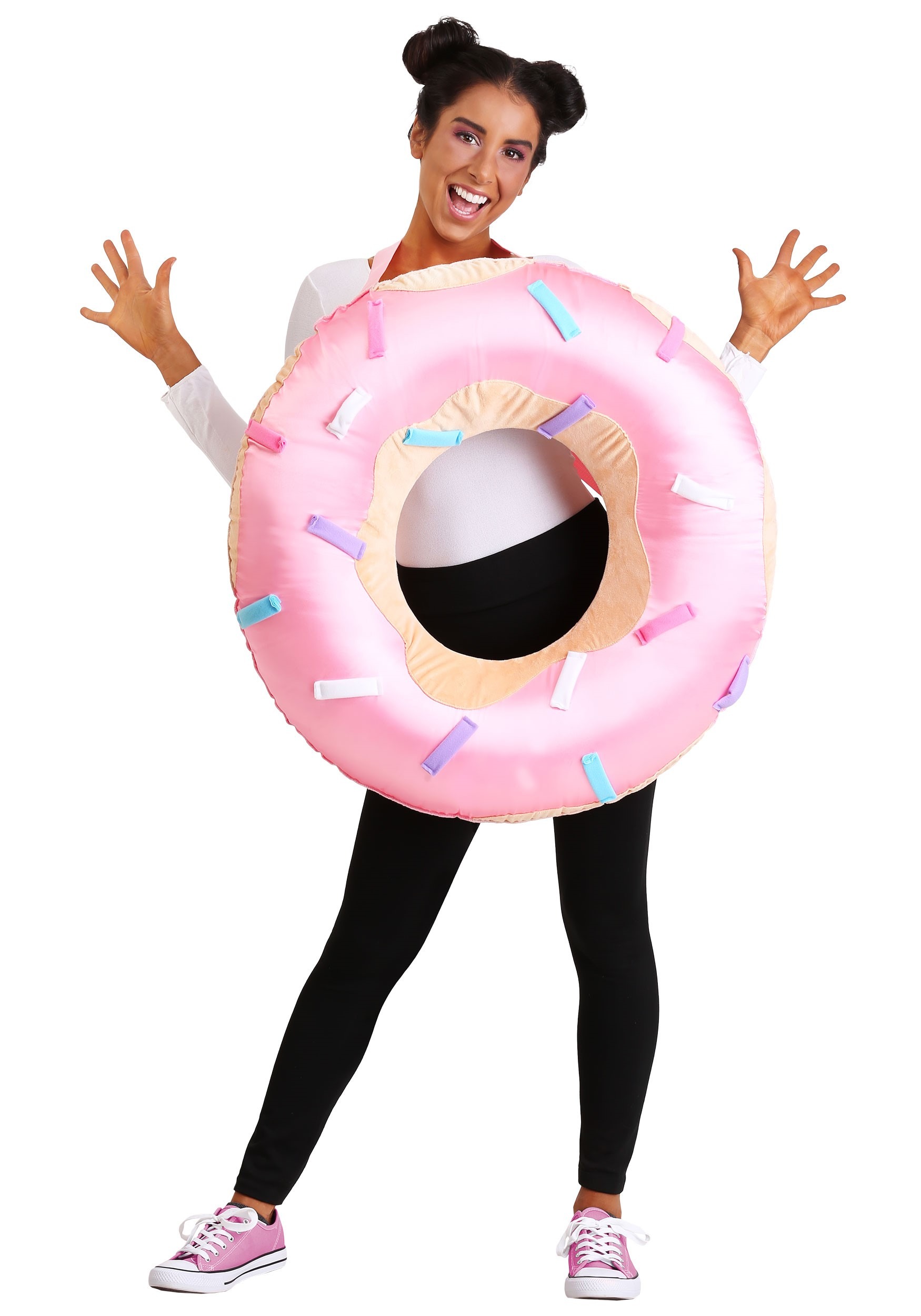This high-quality studio photograph features a realistic, professionally-taken image of a woman in her 20s or 30s against a pure white background. The woman, who has tanned white skin and distinctly European facial features, is depicted with dark hair styled into two buns atop her head. Her eyes are wide open, and she wears a large, open-mouthed smile, revealing her teeth. She appears to radiate enthusiasm with her head slightly tilted to the right and her arms raised, elbows close to her sides, palms forward, and fingers outspread.

Dressed in a long-sleeved white t-shirt, black leggings, and pink Converse-style shoes with visible black ankle socks on her left foot, she exudes a playful and vibrant energy. Around her neck hangs an oversized pink inflatable donut, approximately two feet in diameter, adorned with blue, pink, and purple sprinkles. This donut, complete with a pink strap, appears inflated and serves as a quirky and eye-catching accessory, contributing to the overall whimsical feel of the photograph.